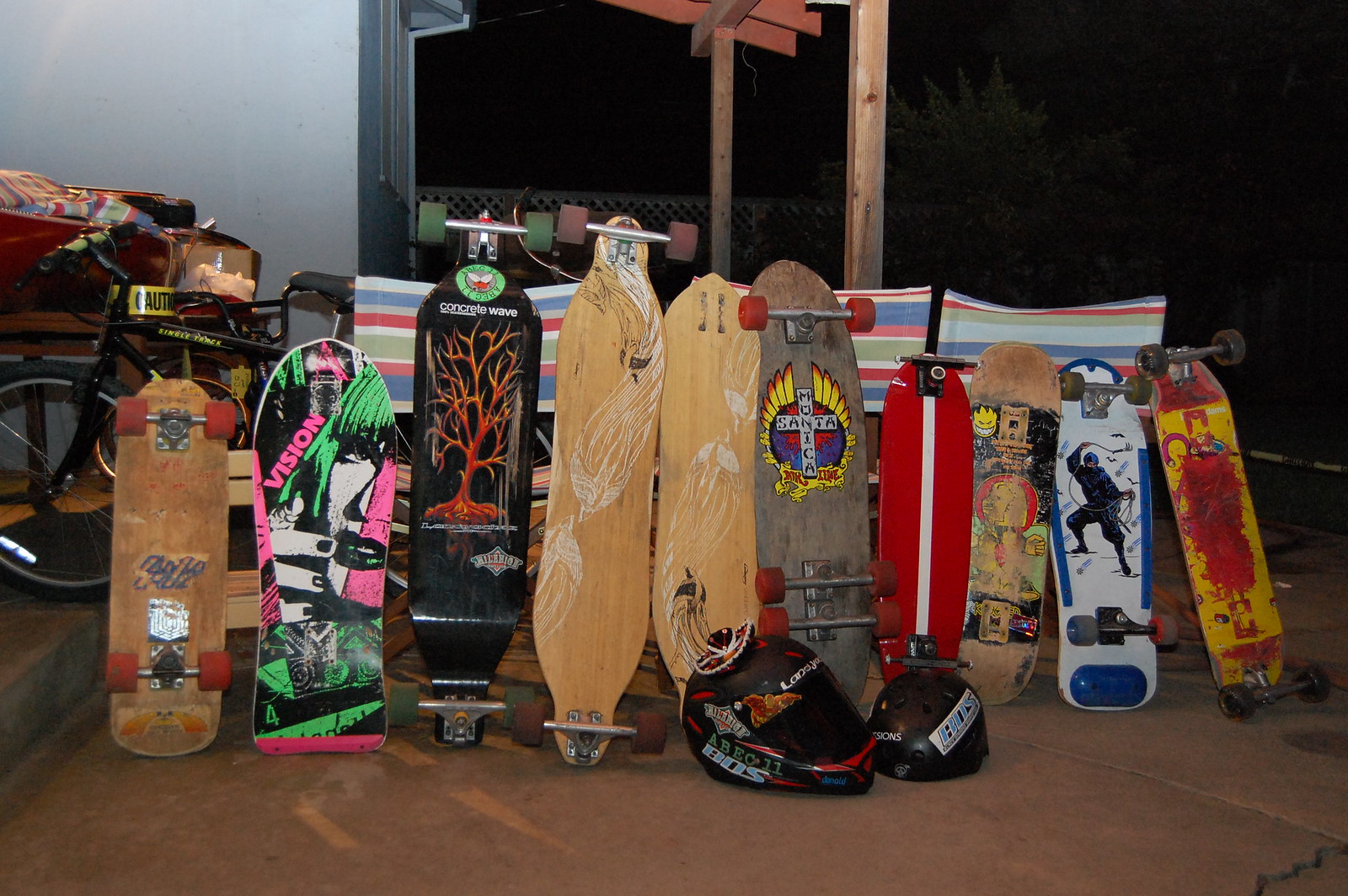Under the cover of night, an intriguing scene unfolds outdoors, featuring a diverse collection of skateboards arranged against a backdrop of a white house, with trees and a criss-crossed metal fence subtly framing the setting. The skateboards, standing on end and showcasing their vibrant underside designs, create a striking display. Noteworthy among them is one skateboard adorned with a vivid red, white, and blue motif, featuring a girl’s face with black and green lipstick, black nails, green hair, and the word "Vision" in pink. Nearby, a black wooden board displays a green logo at the top and a brownish-red and yellow leafless tree. Another skateboard captures attention with an orange, white, and pink palette also bearing the word "Vision." Some boards exhibit raw light wood tones with unique markings, while others flaunt elaborate illustrations, including a black figure wielding a whip, a monochrome tree, a ninja warrior silhouette on a white background, and a red and white striped design. Two black helmets – one detailed with red and white, and the other with blue and white – rest on the ground among the skateboards. To the far left, a black and yellow bicycle adds another layer to this eclectic mix. The scene hints at a concrete or perhaps carpeted patio area, featuring additional objects like striped chairs and enigmatic wooden beams projecting from the structure, creating an overall captivating tableau of skate culture and backyard atmosphere.